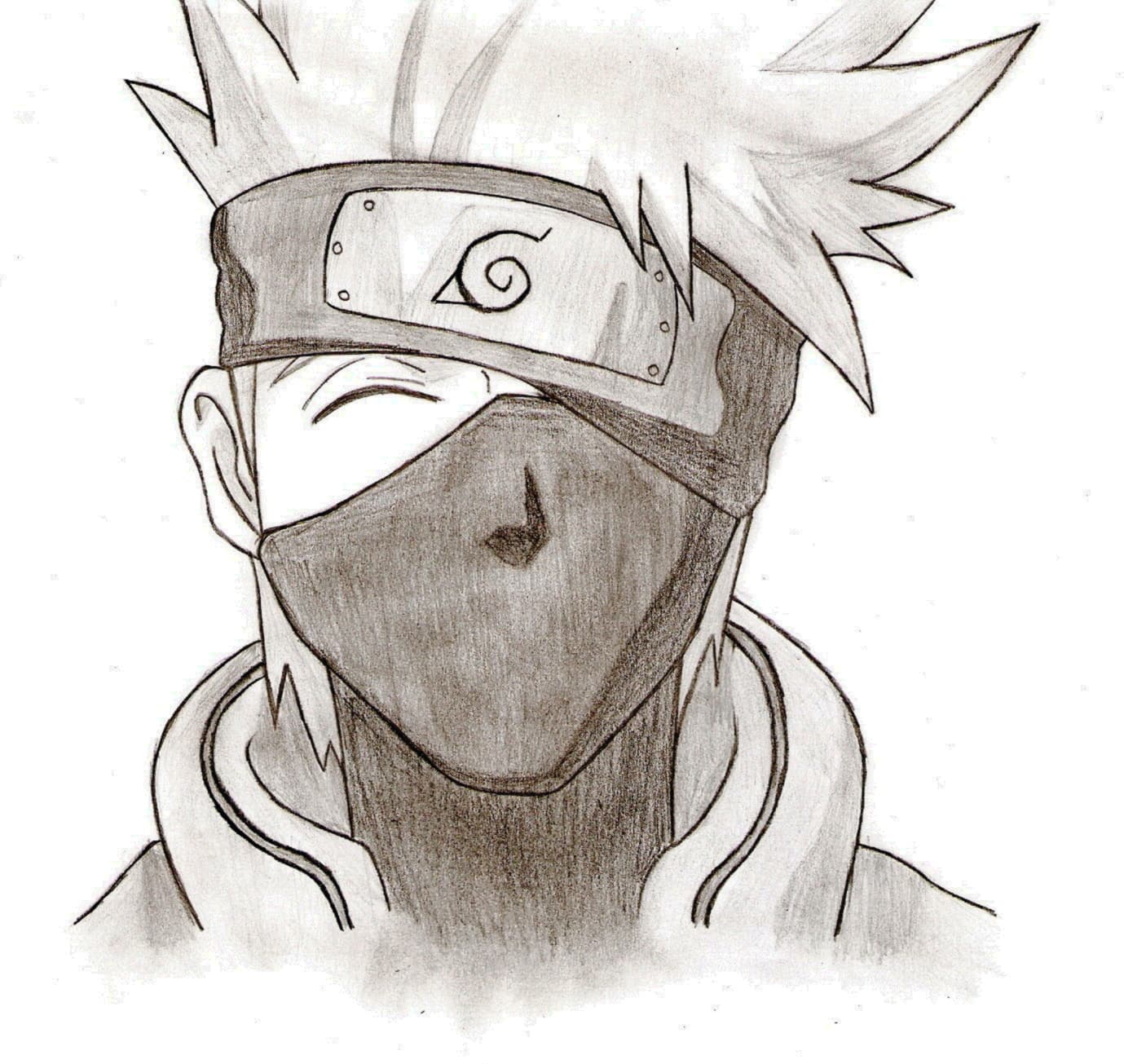This is a detailed pencil sketch of an anime character on white paper, which has some gray specks that appear to be incidental from the drawing process. The character portrayed is a young male with spiky hair and a dark mask covering his mouth, extending down to his neck. He wears a dark, shaded headband with a steel plate on the front, which bears a winding symbol. One of his eyes is visible along with a bit of one eyebrow, giving the impression that he is smiling, while the other eye and ear are obscured by the headband. The character's collar is slightly lighter in shade, marked with a darker line running through its center. The detailed hand-drawn sketch is rendered in a classic Japanese anime style using black, white, and gray tones.